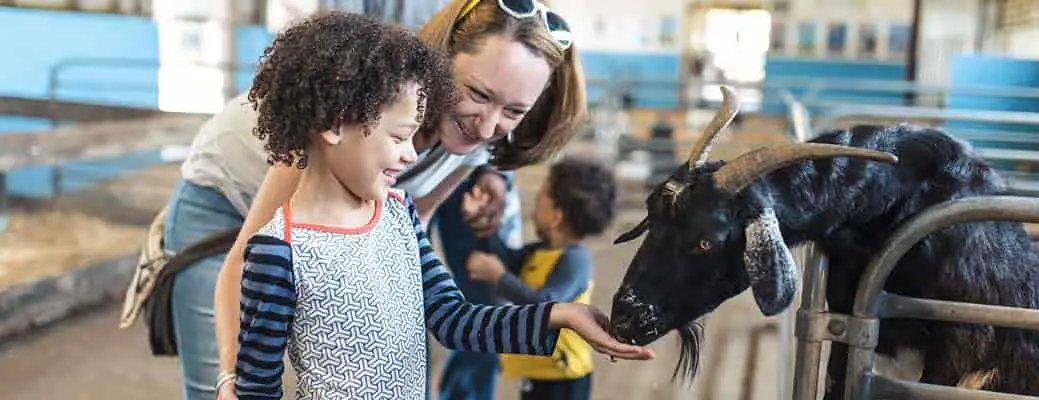In this photograph taken at a petting zoo, a young boy with long black curly hair, who is smiling and wearing a long-sleeved shirt patterned with blue and black circles, is feeding a black goat with yellow-tinged, floppy ears and medium-length yellow horns. The goat, positioned on the right side of the image, leans through the junction of two gates to nibble food from the boy's outstretched hand. Behind the boy, a woman with light brown hair, a white shirt, and blue jeans smiles warmly. She has sunglasses perched on top of her head and appears to be overseeing the interaction with joy. Further back, another child with dark black curly hair and a white shirt with blue sleeves stands slightly out of focus. The background reveals more gates similar to the one the goat is leaning through, along with a teal-colored wall that adds a vibrant touch to the scene, giving the impression of an indoor-outdoor enclosure typical for a petting zoo.